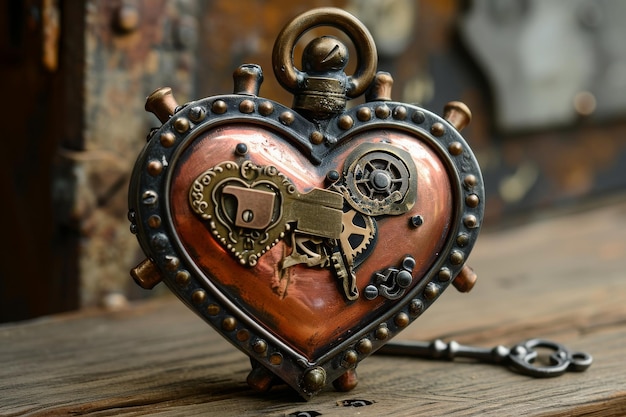This color photograph captures a detailed steampunk-inspired scene featuring a heart-shaped metallic lock adorned with intricate gear patterns. The heart lock is predominantly bronze with a burnt orange core and is outlined with numerous raised brass circles. At the top, it features a brass circular hook, suggesting it could be hung or suspended. The lock sits on a rustic wooden table, with a matching old-fashioned key lying just to its right. The background, while out of focus, hints at a blend of natural textures and colors, possibly suggesting an indoor setting with elements resembling aged wood and metal. The intricate details and patina give the overall image a rich, vintage aesthetic, emblematic of modern steampunk artistry.